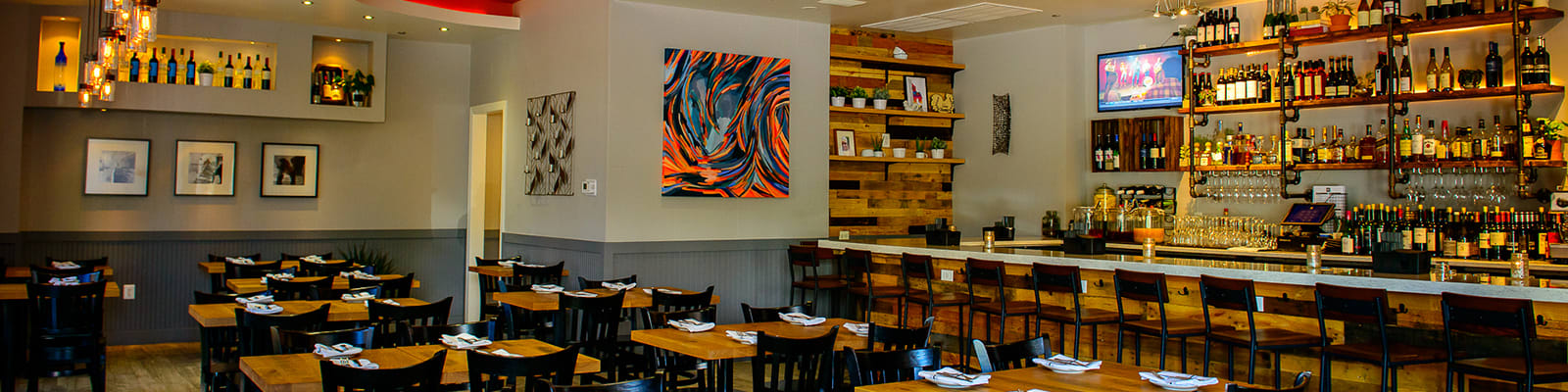This photograph captures the interior of a restaurant-slash-sports bar before it opens. Dominating the scene is a long bar lined with ten tall stool chairs, each featuring a backrest, ready to accommodate patrons. Behind the bar, an array of cabinets showcase an extensive selection of liquors and wines, adding a sense of opulence to the scene. Mounted above the bar is a TV screen, likely for entertainment during service hours.

The seating area is composed of seven brown wooden tables, each accompanied by four black chairs, neatly arranged and set with napkins and silverware, indicating preparedness for guests. The floor appears to be wooden, enhancing the warm and inviting ambiance of the space.

Decorating the walls are several pieces of art: a large abstract painting characterized by swirls of orange and various shades of blue, three framed pictures of people, and another intriguing artwork that appears to depict knives. Bottles of alcohol are also prominently displayed on another wall, reaching high above. In the background, the route to the bathrooms is visible, completing the layout of this well-appointed establishment.